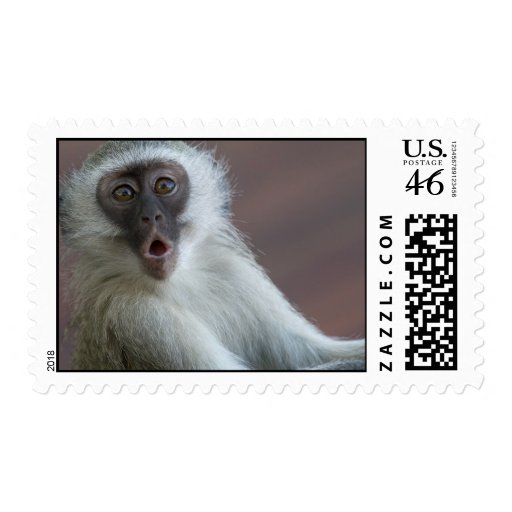The image is of a horizontally oriented United States Postal Stamp with a crisp white background and a ridged pattern along its edges. Dominating the left side of the stamp is a photograph of a monkey with dense white fur and a dark brown face. The monkey's large, golden yellow eyes with black pupils are wide open in surprise, and its mouth forms an "O" shape, revealing a hint of red that suggests its tongue. To the right of this striking image, "Zazzle.com" is written vertically from bottom to top, followed by a 2D barcode below. In the upper right corner, the text "U.S. Postage 46" is prominently displayed, with a black diagonal line striking through the number 46. The year "2018" is subtly inscribed to the left of the monkey image.